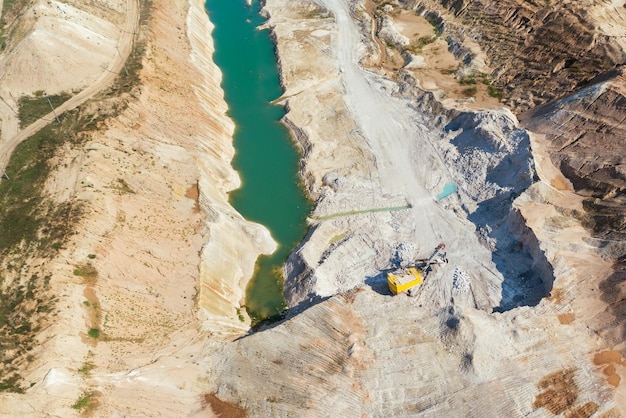This aerial view captures a rugged rock quarry characterized by steep, smooth, and brown sandstone-like cliff walls on both the left and right sides. Sparse vegetation and patches of short green grass are apparent, growing at various levels along the cliffs, especially on the left. A distinctive long, skinny pond with still, turquoise-green water runs through the center of the quarry, framed by the rocky terrain. On the right side, there is an intriguing blue-cast formation, possibly a chunk of ice. Notably, a yellow piece of excavation equipment with a long neck, likely a crane, is situated prominently at the bottom of the quarry. A dirt road, lined with light or power line poles, traces the top left edge of the quarry. The scene is bathed in bright sunlight, adding vibrancy to the lack of human presence, making the man-made yellow structure even more conspicuous amid the natural landscape.